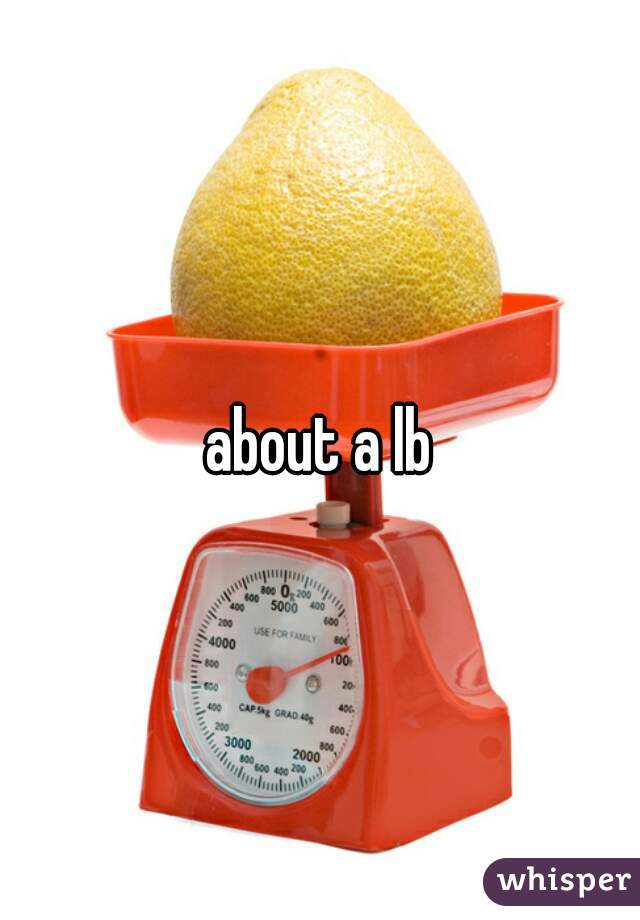This image features a bright red, old-style plastic dial kitchen scale set against a plain white background. The scale showcases a classic design with a white face displaying measurements in grams, ranging from 0 to 5,000 grams, with a red needle indicating a weight close to 900 grams, or about one pound as denoted by superimposed white text with a black outline. The scale's design includes rounded edges and a dome-like structure on top, which forms a bowl holding a glossy, bright yellow fruit that resembles an Asian pear or some type of citrus. The fruit's surface reflects light, enhancing its vibrant, shiny appearance.